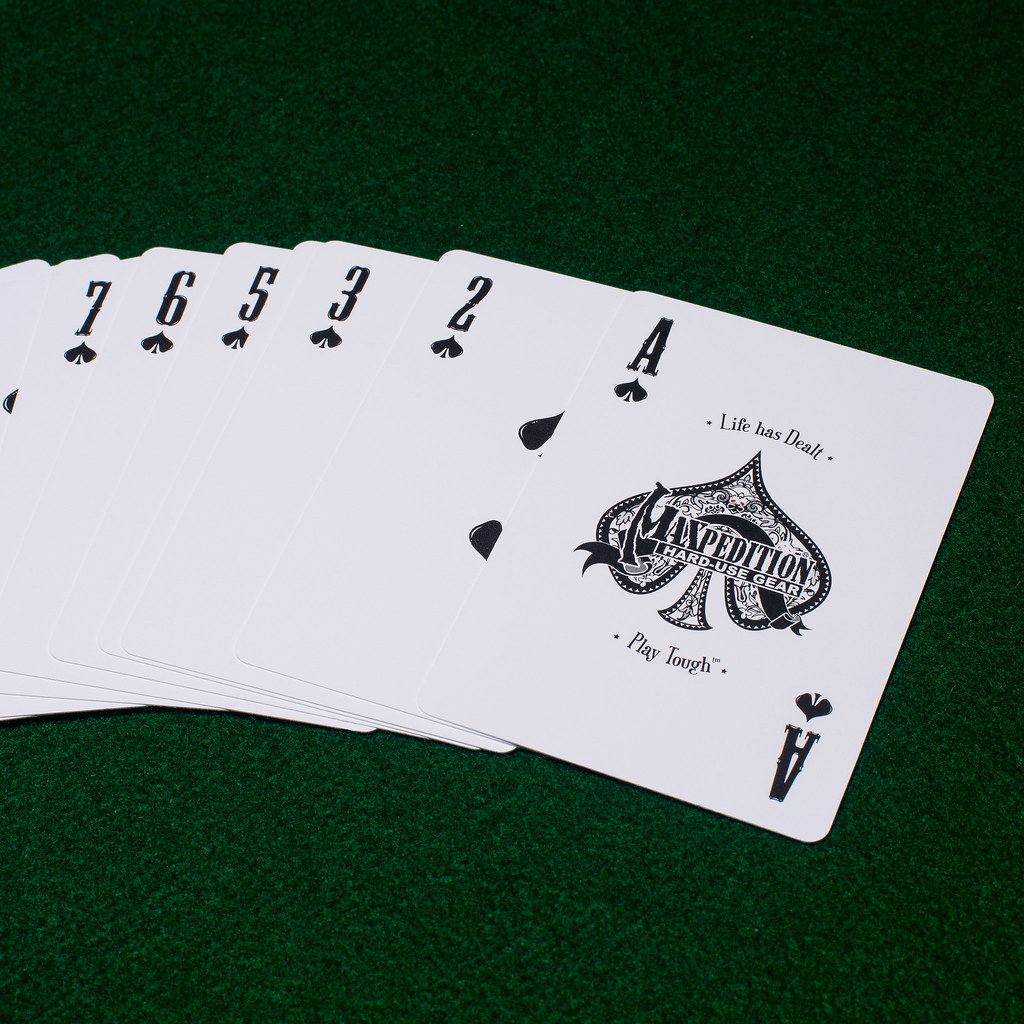A high-resolution close-up photograph captures a pristine hand of playing cards meticulously arranged on a luxurious, professional-style poker table. The table features an elegant, rich green felt surface typically seen in high-stakes poker settings. Dominating the image are seven brand-new, unblemished playing cards, each one a spade, laid out from right to left. The sequence shows an Ace of Spades, Two of Spades, Three of Spades, partially obscured Four of Spades, Five of Spades, Six of Spades, and Seven of Spades. The Ace of Spades stands out with its intricate design: within the spade symbol is the branding "Maxpedition, Hard Use Gear" along with the phrase "Life Has Dealt, Play Tough," adding a unique touch to the card's traditional look. The fine details in the spade's design, combined with the impeccable condition of the cards, contribute to a clean and sophisticated visual presentation.